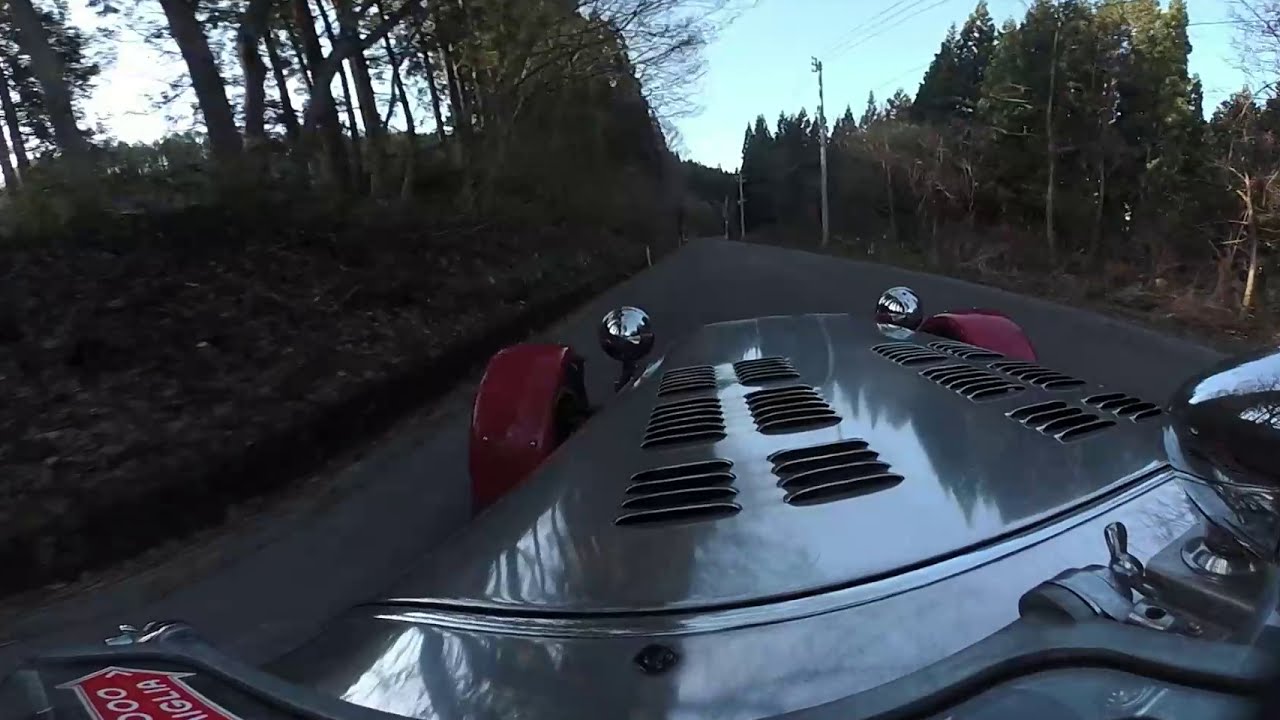This detailed photograph captures an older, souped-up car driving down an otherwise empty, single-lane country road surrounded by a mix of dry and green-leaved trees and an overhead stretch of clear blue sky. The vehicle, a meticulously restored model from the 1940s or 50s, is coated in a shiny metallic gray paint and flaunts distinctive features. It boasts 12 vents arranged symmetrically on the top of its black bonnet, with six on each side. The front end is accented with oversized, burgundy fenders and matching bumper guards, along with pop-up headlights that add to its vintage allure. Visible from inside the car, the front wheel also sports the same striking red hue. The image conveys a sense of a leisurely Sunday drive, perhaps en route to a car show, highlighting the unique charm and extensive work put into modifying this classic automobile.